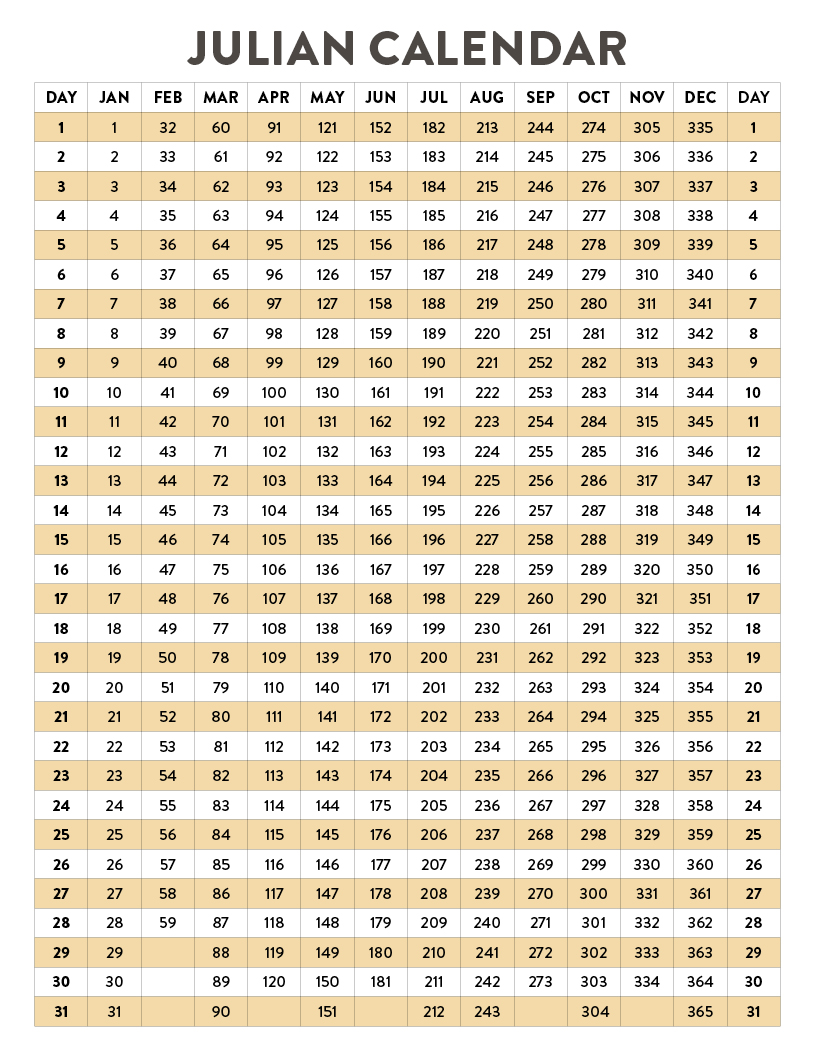This image features a detailed Julian calendar. The words "Julian Calendar" are prominently displayed in bold letters. The calendar is designed with a blend of white and brown lines, consisting of 31 rows and 14 columns. Each row represents the days from 1 to 31, while the columns represent the months from January to December. 

The calendar allows you to determine the day of the year by cross-referencing the date with its corresponding position. For example, August 14th marks the 226th day of the year, while April 18th is the 108th day. December 31st, being the last day of the year, is noted as the 365th day. This comprehensive layout enables users to quickly identify the specific day of the year for any given date.